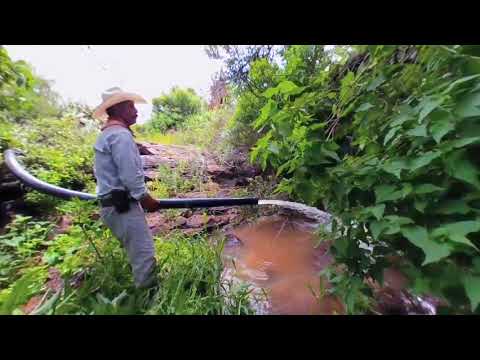The image depicts a man standing in a lush, heavily vegetated area by a muddy stream or pond with reddish-brown water. He is wearing a straw cowboy hat, a light denim shirt and pants, and a belt that appears to have a smartphone or pouch attached to it. The man stands in tall green grass and is holding a long black hose from which water is spraying into the rocky, muddy puddle before him. Surrounding the man and the water are dense green leaves and vegetation, while the background features a whitish sky. The scene is saturated with the earthy tones of the muddy water and the vibrant greens of the vegetation, with the man’s attire providing a contrasting light hue.